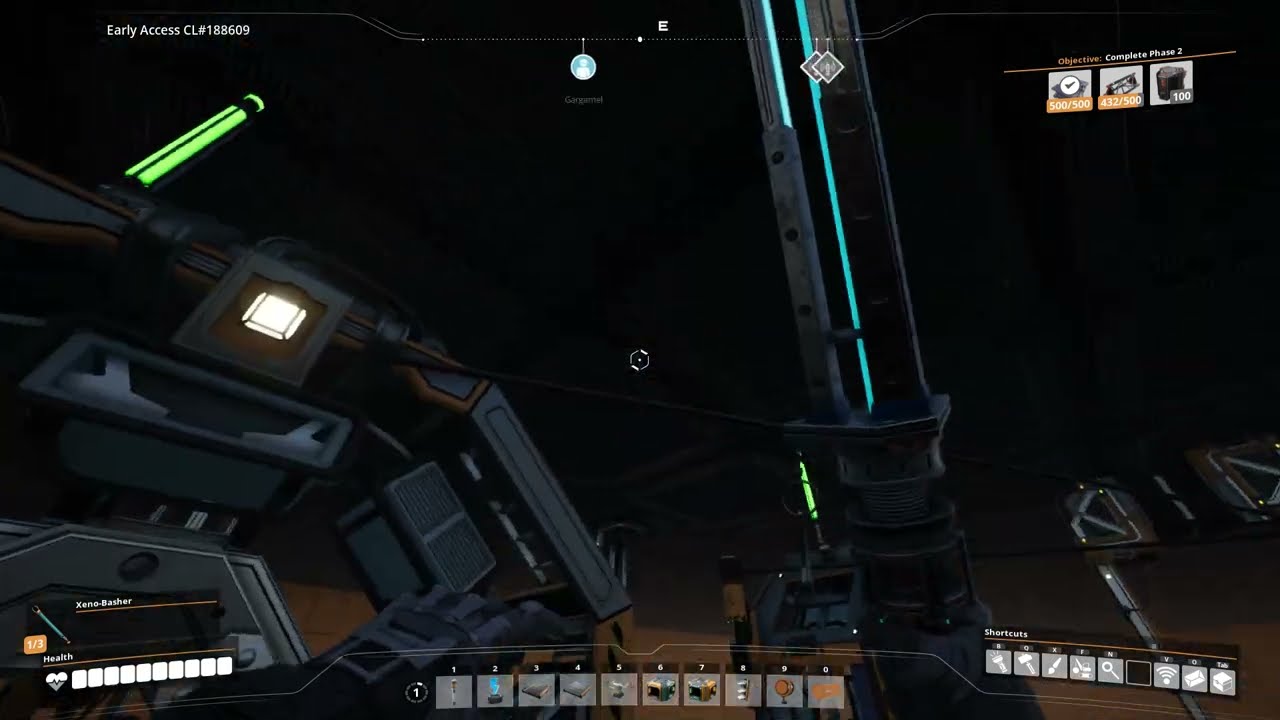The image is a dark theme, likely a screenshot from a video game, showcasing an interface with a black background. The main visual element in the center resembles a long cylindrical, weapon-like object, with two blue lines extending vertically from it, possibly positioned within the confines of a ship or shuttle. Surrounding the central figure, numerous icons and menu elements populate the screen. 

In the upper right-hand corner, there are three icons alongside text that reads "Objective: Complete Phase 2." The upper left-hand corner contains text that says "Early Access CL Number 188609." The bottom section of the screen features various small gray squares with white icons, likely representing different objects or items within the game. These icons form a digital control panel overlay with selectable menu items. The lower right has a section labeled "shortcuts," while the bottom center shows additional icons. The overall aesthetic includes teal lighting accents along the ship's frame, emphasizing a sci-fi atmosphere. In the middle, there's also a small circular crosshair indicating the ship's heading.